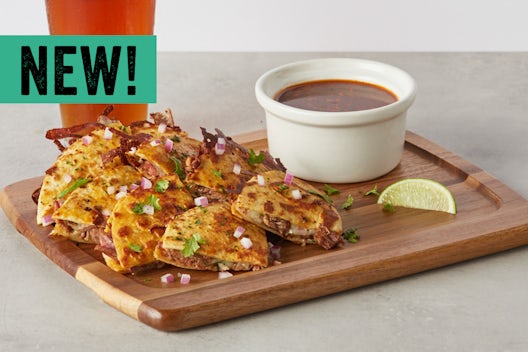The image is an advertisement for a restaurant, showcasing a new menu item. It features a rectangular, dark wooden serving tray with text reading "NEW" in black letters on a green background in the upper left corner. The tray holds eight pieces of golden-brown quesadilla, each filled with ground beef and garnished with diced red onions and parsley flakes. The quesadillas are arranged diagonally in pairs. To the right of them is a small white cup with a reddish condiment, accompanied by a single slice of lime positioned in front of the cup. In the background, a red drink can be partially seen but remains indistinct. The vibrant display of the food, toppings, and accompaniments creates a visually appealing and inviting presentation.